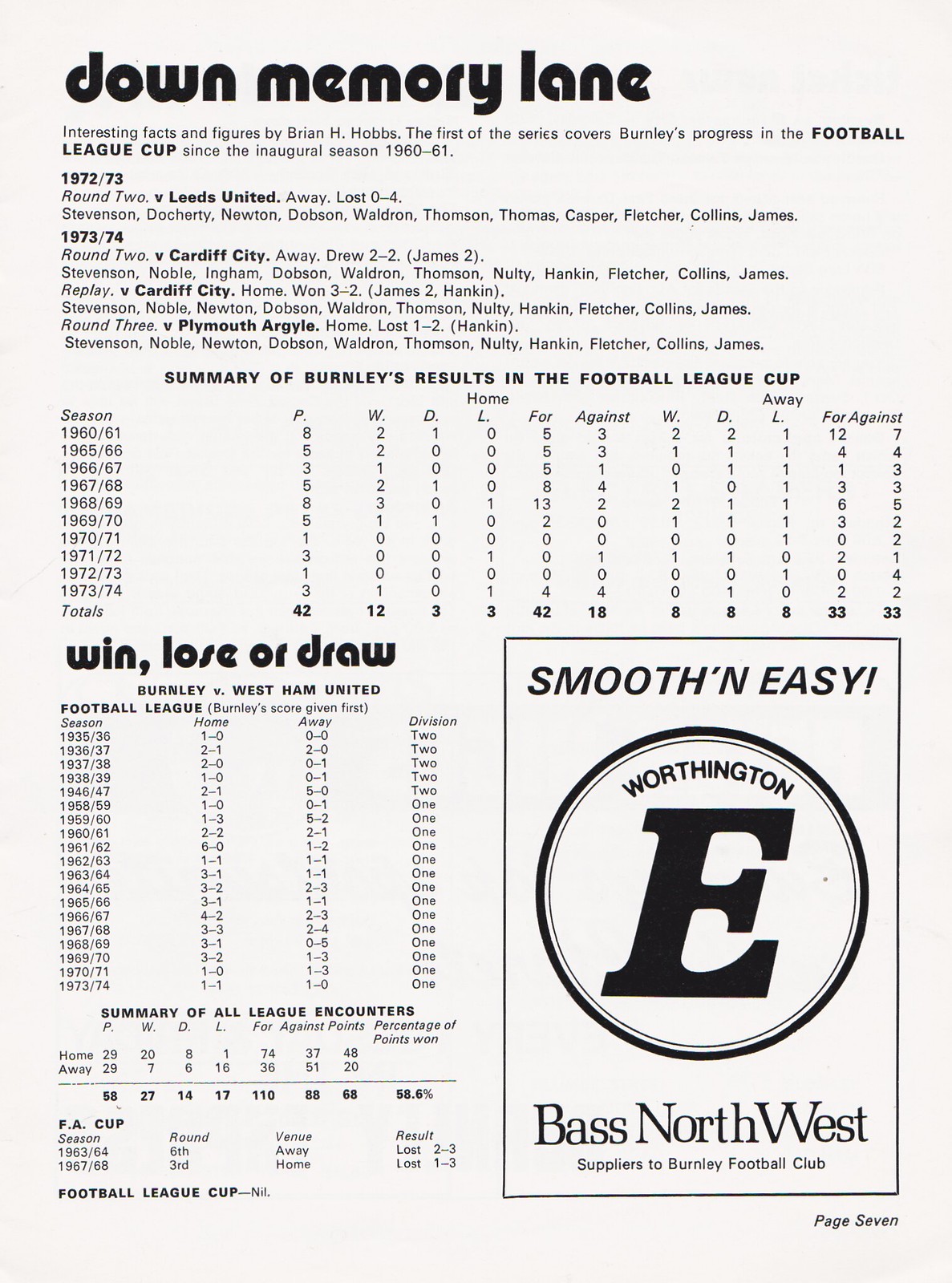The image depicts a vertical, rectangular page with a clean white background and black text. At the top, bold letters read, "Down Memory Lane," with an introduction by Brian H. Hobbs. This page is part of a series detailing Burnley Football Club's history in the Football League Cup, focusing on the seasons from 1960-61 through to the early 1970s. 

The primary content includes match histories, specific results, and player line-ups, such as the 1972-73 Round 2 away loss to Leeds United (0-4) and the 1973-74 Round 2 draw away to Cardiff City (2-2), followed by a home replay (3-2). Detail is given to various encounters with clubs like Cardiff City and Plymouth Argyle. 

The page is structured into multiple columns summarizing Burnley's performance, listing wins, losses, and draws across different seasons and against various opponents within these competitions.

At the bottom left corner, the text reads "Win, Lose, or Draw" and "Summary of All League Encounters," while the bottom right corner features "Smooth and Easy, Worthington E. Bass Northwest Suppliers to Burnley Football Club" and "Page 7." This detailed overview captures the statistical and narrative essence of Burnley's past performances, making it a historical tribute to the club's legacy in the Football League Cup.